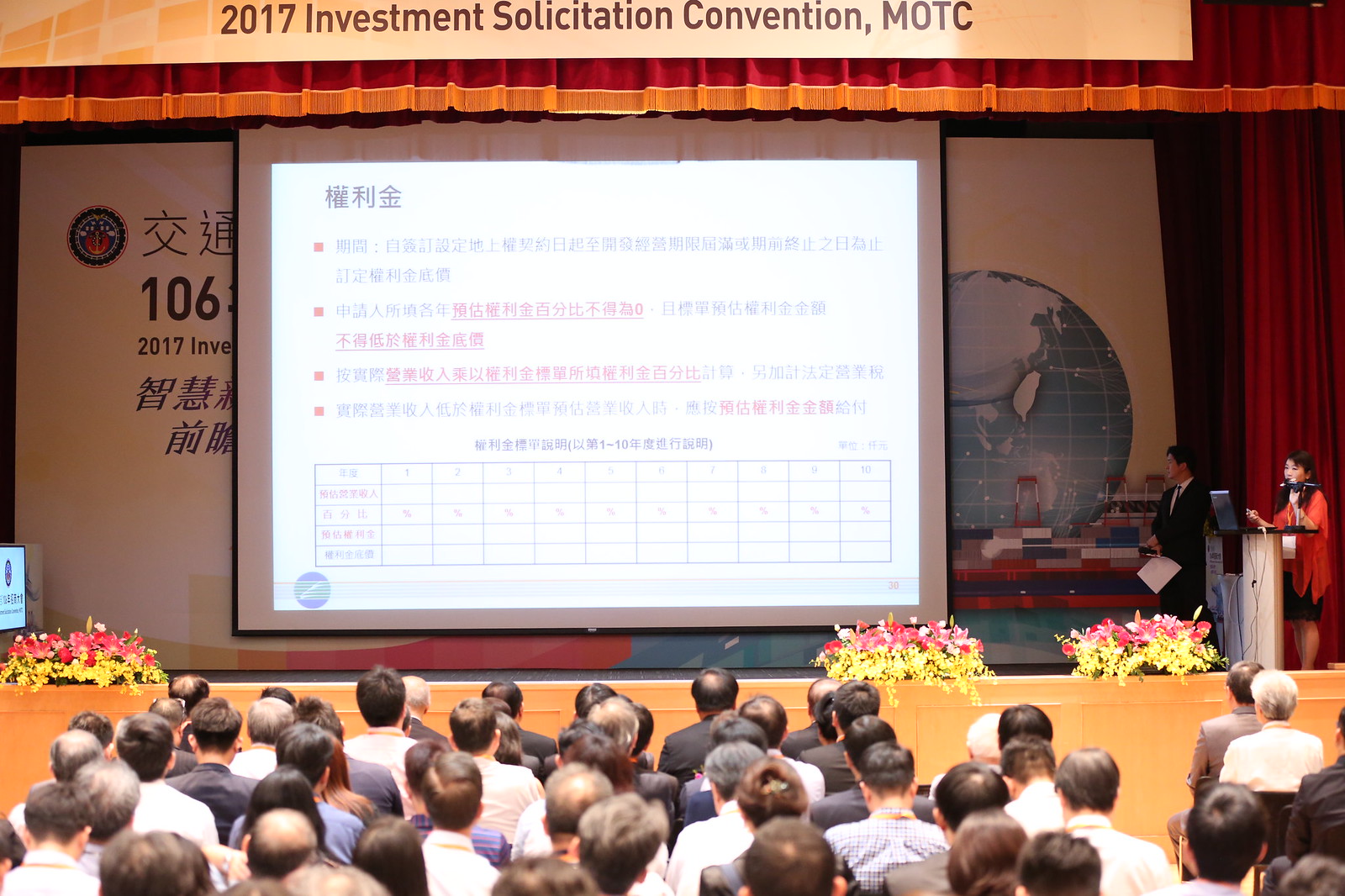The image captures a scene from the 2017 Investment Solicitation Convention, MOTC, presumed to be held in China. At the center stage, a large projector screen displays a PowerPoint presentation with Asian characters and a graph chart. Above the screen, a partially visible sign showcases a globe. To the right of the screen stand a woman and a man beside a podium. The woman, who is speaking into a microphone, is dressed in a red jacket, black skirt, and white shirt, while the man next to her wears a black suit with a white collared shirt and tie. The foreground reveals the backs of the audience members, varied in age and gender, many of whom are dressed in suits or collared shirts. Red and green floral arrangements decorate the front of the stage, adding a touch of color to the professionally set scene.